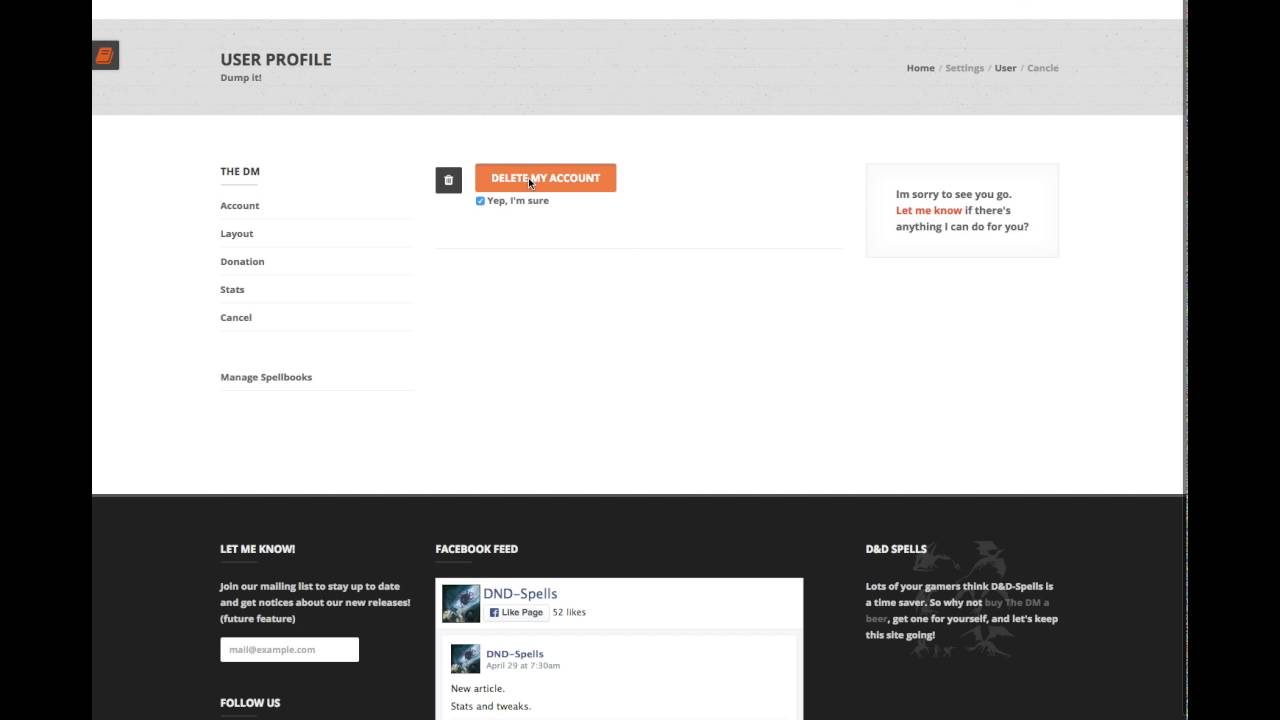The image depicts a user interface with a predominantly grey background. The screen includes several elements: a user profile section, options to navigate home, settings, user management, and conical. There's also a direct messages (DM) area, account settings, layout configurations, donation options, and statistics. The interface offers a "Cancel" button, access to "My Soapbox," and options to transfer content or delete the account.

Additionally, there is a mailing list invitation section encouraging users to join in order to stay updated on new releases. The text overlay includes a message: "Let me know if there's anything I can do for you." The aesthetic incorporates white backgrounds with a black vertical border on the far left and right edges of the page. The interface features content on philosophy and Dungeons & Dragons (DnD) spells, which appear to be popular among users. Article sections and various page elements are also highlighted, contributing to a complex and busy layout.